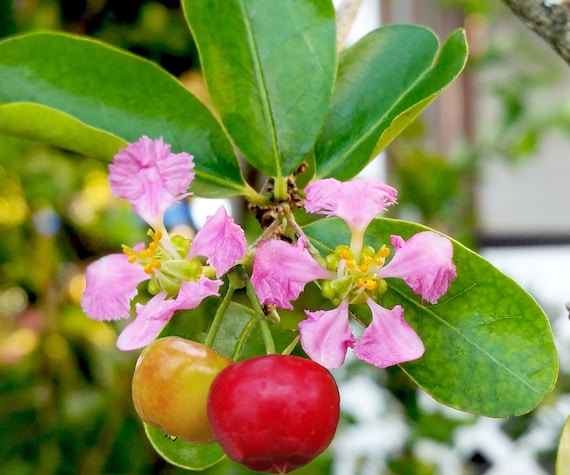In this daytime color photo, the focus is on a branch from a fruit tree adorned with both flowers and fruit. The foreground prominently features two dangling fruits, one a fully ripened bright red, the other a yellow-orange hue, both about the size and appearance suggesting they might be cherries or possibly small crab apples. These fruits hang beneath a cluster of five delicate pink-lilac flowers, each embodying a rosy hue, with visible yellow pollen sacs. The leaves are large, smooth, oval, and a deep green, evoking a tropical aesthetic. The background is a blur of green foliage, hinting at a garden or yard, with a white, lattice-style trellis visible in the lower right, adding a structural element that suggests the photo might be taken in front of a house. A smudge of blue in the corner contrasts subtly against the greenery, possibly reflecting the sky or a nearby object.